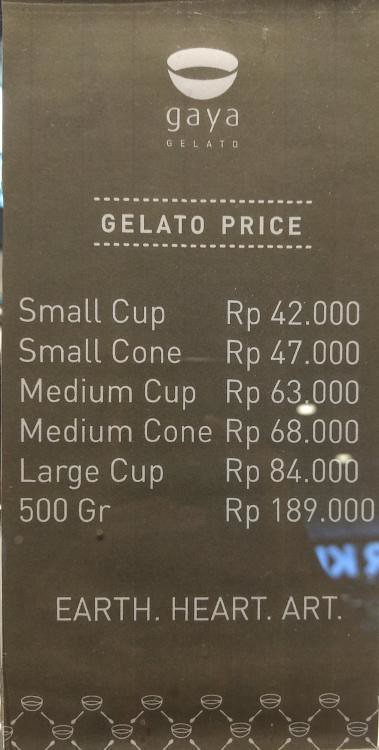In this image, we see a zoomed-in view of a menu from Gaia Gelato. The menu predominantly features a black background with white text, listing the prices in Indonesian Rupiah (RP). At the top of the menu, the Gaia Gelato logo includes a small gelato cup. The pricing details are neatly centered, indicating:

- Small cup: 42,000 RP
- Small cone: 47,000 RP
- Medium cup: 63,000 RP
- Medium cone: 68,000 RP
- Large cup: 84,000 RP
- 500 grams: 189,000 RP

The phrases "Earth. Heart. Art." are capitalized and punctuated with periods beneath the price listings. A light blue reflection, likely due to the glass covering the menu, is visible, suggesting an indoor setting. The background design incorporates gelato cup patterns forming a grid at the bottom. Additional elements, such as a grey standing sign with white font, and a faint forest reflection in bluish-white lettering, contribute to the ambience of a gelato shop. This detailed visual and textual description cohesively presents the image of the menu.